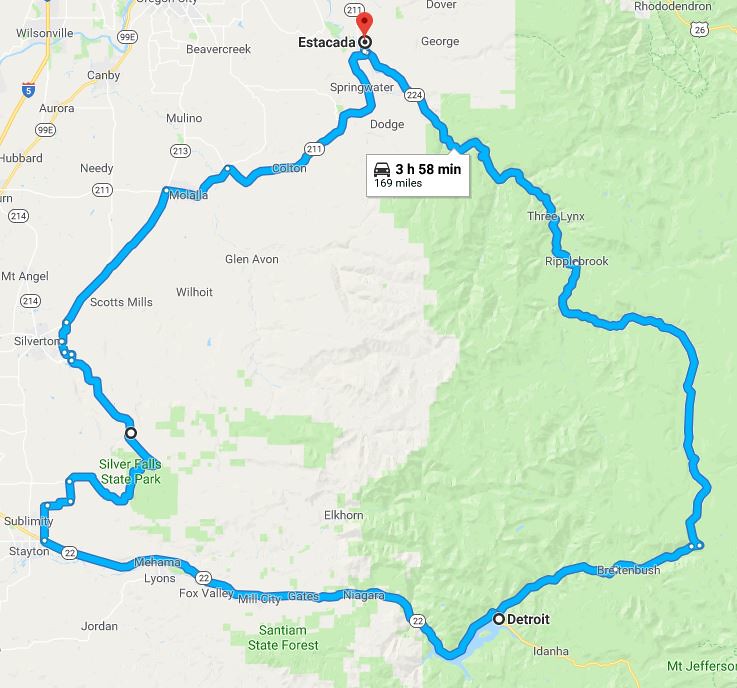This detailed caption is of a screenshot from an online map, likely from Google Maps, showcasing two possible routes between Detroit and Estacada. The map's right side is predominantly green, indicating a mountainous and forested area, while the left side is grayer and flatter. The primary route, depicted in turquoise blue, spans 169 miles and is estimated to take three hours and 58 minutes by car. It follows a zigzag path that almost forms an oval shape. Key landmarks along the route include Snow White, Ripperbrook, Three Links, Cotton, Morajala, Silverton, Silver Falls State Park, Subway, Slayton, Magna Linos, Fort Malley, Mill City, Gates, and Niagara. The map also displays nearby towns such as Aurora, Hubbard, Canby, Wilsonville, Beaver Creek, Molino, Springwater, Dodge, George, Dover, Rhododendron, Needy, Mount Angel, Scotts Mills, Wilhoit, Glen Avon, and Elkhorn. Notable geographical features include Santiam State Forest and Mount Jefferson. The destination, Estacada, is marked with a red pin at the top, while the starting point, Detroit, is located at the bottom right. Additionally, the map indicates a general southward positioning of Seneton State Forest.